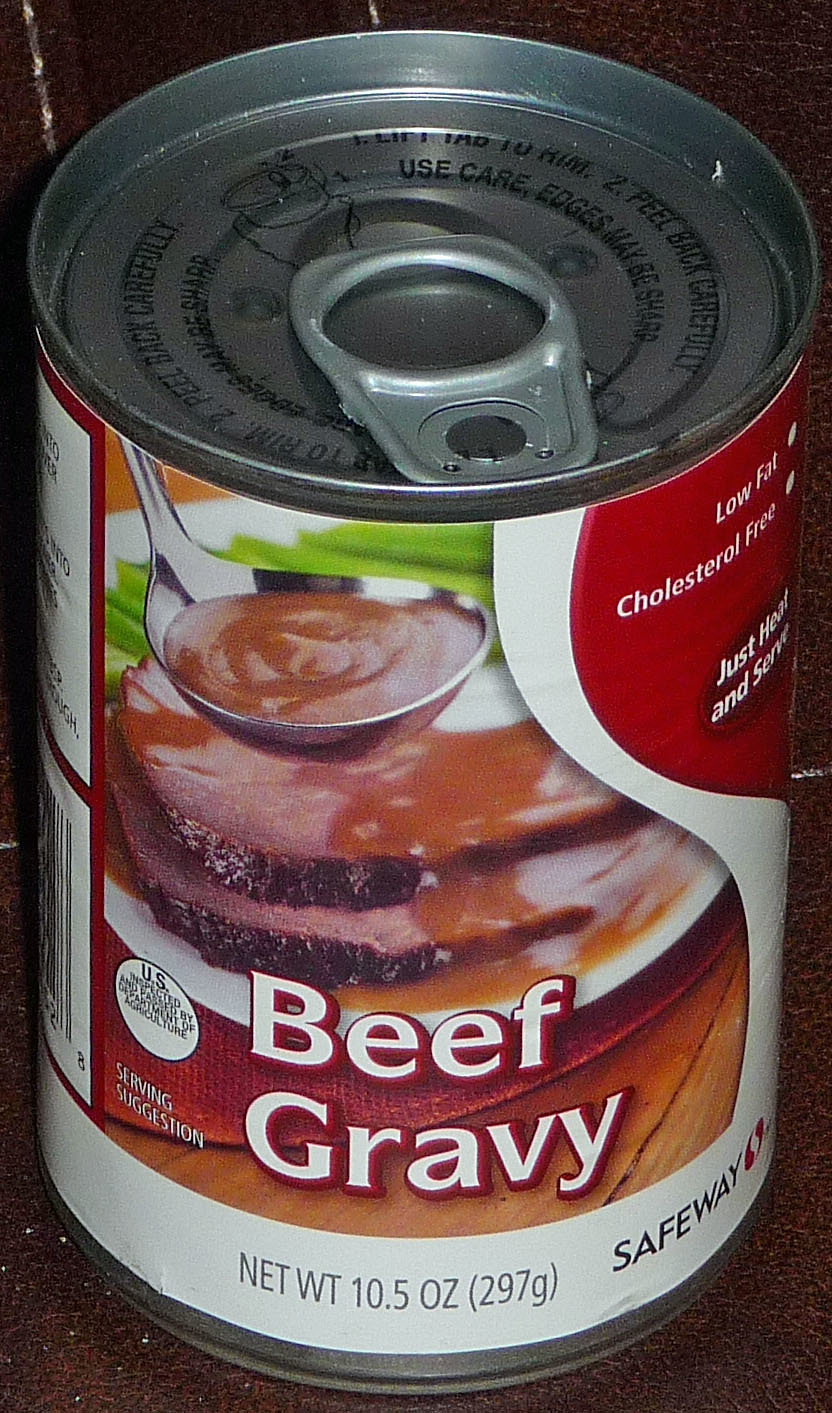This is a close-up photograph of a can of Safeway brand beef gravy, prominently featuring its distinctive design. The can is round with a silver aluminum pop top, designed for easy opening without a can opener. The label is predominantly white with a red section snaking around the back, making it visually striking. The label includes a detailed image of brown gravy in a spoon being drizzled over two slices of meat, which appear to be ham, accompanied by a hint of green celery in the background. The text on the can clearly reads "Beef Gravy," along with important product details such as "net weight 10.5 ounces (297 grams)," "low-fat," "cholesterol-free," and "just heat and serve." The top of the can also features some black writing, adding to the intricate design of the packaging. The entire setup is positioned on a brown table, highlighting the packaging's aesthetics.